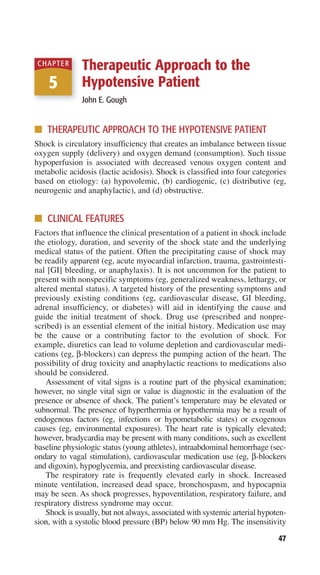The image is a photograph of a text document, specifically a page from a medical book or magazine. The page, oriented in portrait, prominently features the headline "Therapeutic Approach to the Hypotensive Patient" in red text at the top. The upper left corner displays a rectangular graphic with a gold bottom and a red arc at the top, containing the word "Chapter" and the large white number "5." The body of the page consists of two main sections, each starting with a red title accompanied by a square gold bullet point. 

The first section is titled "Therapeutic Approach to the Hypotensive Patient," and it includes a paragraph discussing the definition of shock, which is described as a circulatory insufficiency that leads to an imbalance between tissue oxygen supply and demand. It mentions that this insufficiency results in decreased venous oxygen content and metabolic acidosis, and categorizes shock into four types based on etiology: hypovolemic, cardiogenic, distributive (including neurogenic and anaphylactic), and obstructive.

Below this, the second section is titled "Clinical Features" and contains three paragraphs detailing the vital signs and clinical features used to assess the condition of a hypotensive patient. The text is in black on a white background, typical of a print publication, with the overall style resembling that of a formal medical document. The page number 47 is located at the bottom right corner.